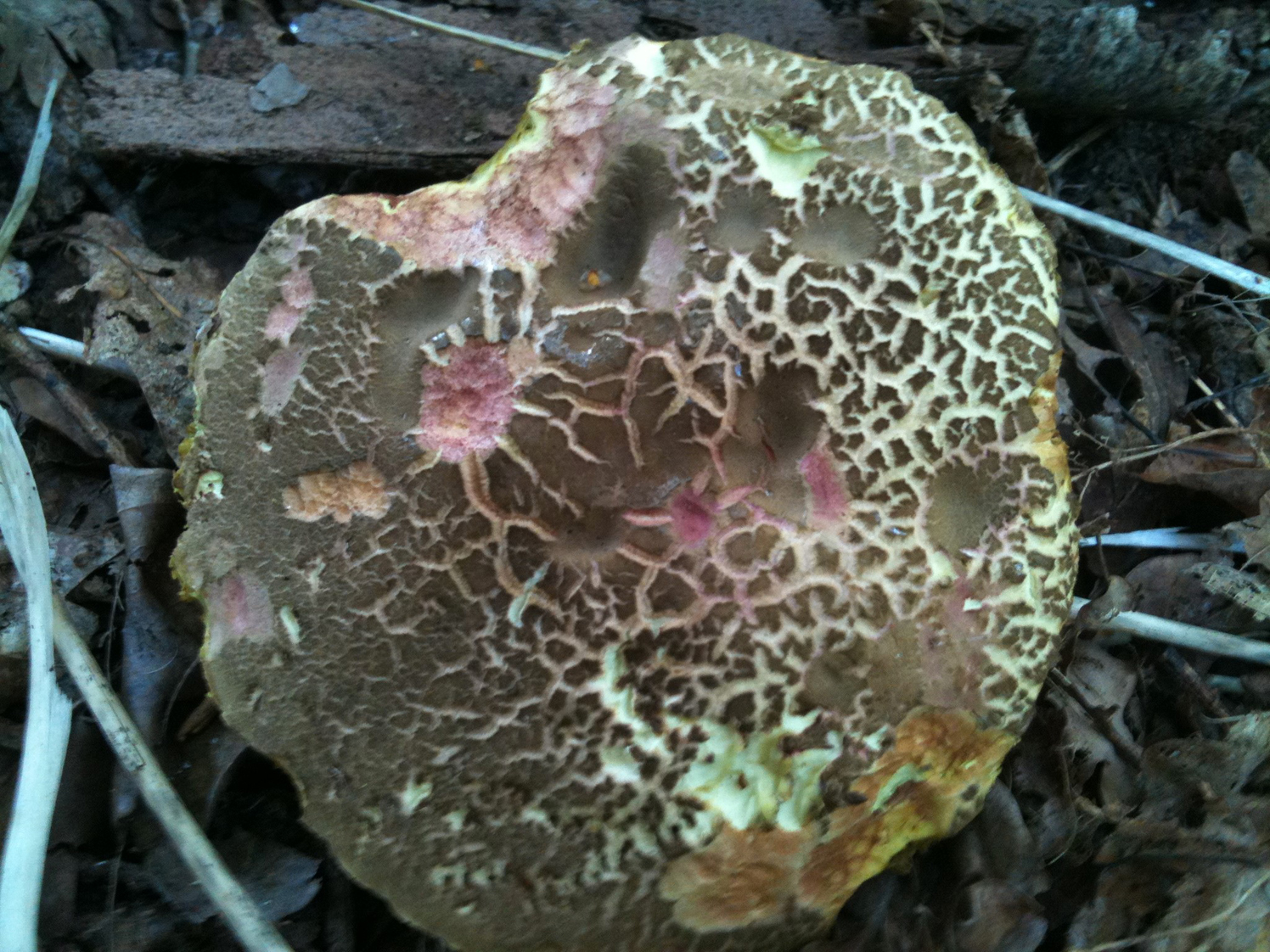A detailed black-and-white overhead photograph captures a single, large mushroom amid a forest floor littered with decaying debris. The mushroom, occupying the majority of the frame, features a medium brown cap with intricate white crack lines, indicating it is drying and starting to separate. The cap is irregularly shaped, resembling more of a cookie than a typical toadstool. A significant portion of the upper left corner appears to have been nibbled away, revealing the mushroom's distinctive fleshy pink interior. The surrounding forest floor is scattered with dark brown leaves, gray decaying stems, and pieces of wood or bark, adding texture and depth to the scene.